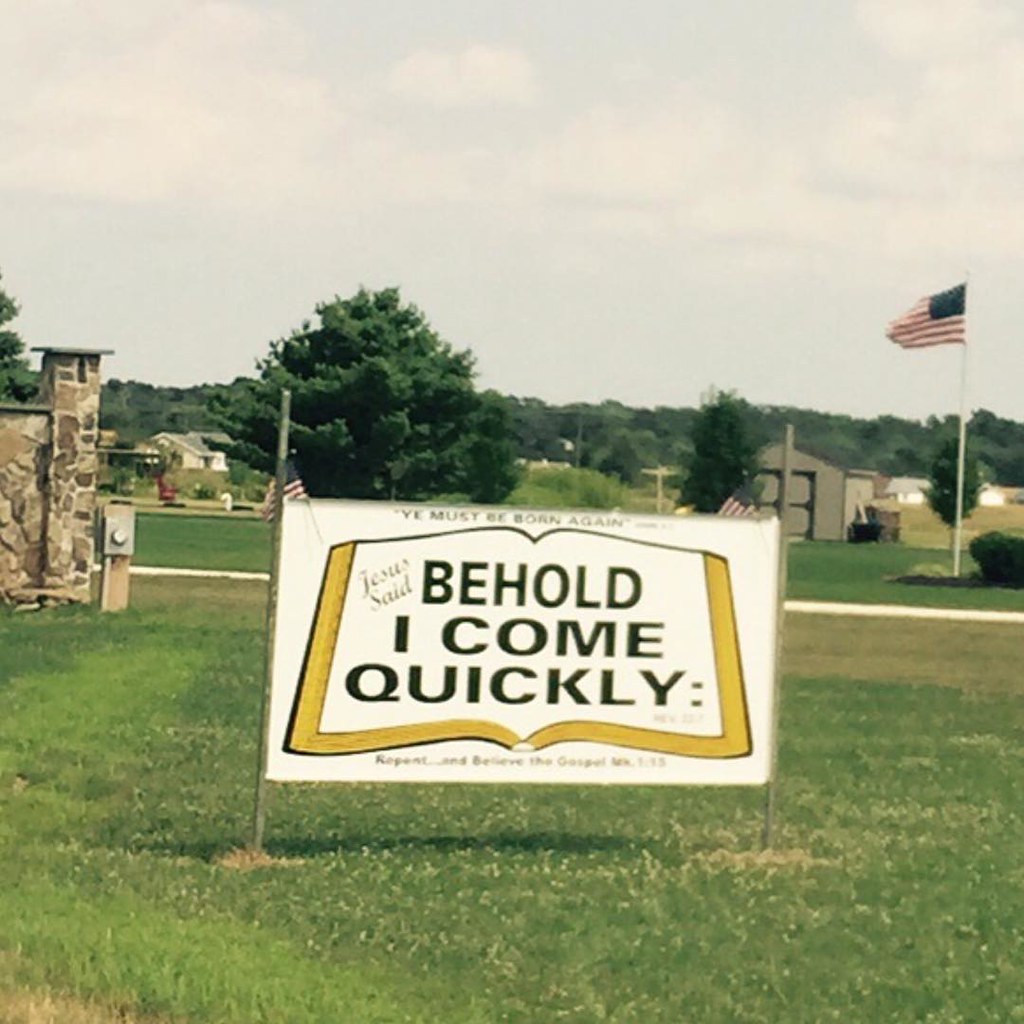This photograph captures a historical-looking sign situated in what appears to be a rural area, potentially a school zone or a military base, judging by the surroundings and context. Prominently displayed on the sign are the words "You must be born again," written in a bold and commanding font. Below this declaration is an illustration of an open Bible, positioned at its centerfold. The Bible's pages are blank except for a prominently displayed text: "Jesus said, 'Behold, I come quickly'." The phrase "Jesus said" is elegantly inscribed in cursive script, while "Behold, I come quickly" is rendered in bold, making it strikingly noticeable. Unfortunately, additional text below this message is too blurry to discern.

The style and graphic design of the sign suggests that it dates back to the 1980s, with elements that may remind one of mid-20th century war propaganda posters. Surrounding the sign, an American flag waves in the background, symbolizing a sense of patriotism. The landscape features vast expanses of green grass, fields, and some trees, enhancing the rural ambiance of the scene. A few buildings can be seen in the distance, indicating that they might all belong to the same expansive property, possibly several acres in size. The overall atmosphere evokes a nostalgic and somewhat solemn mood, reflective of its era.